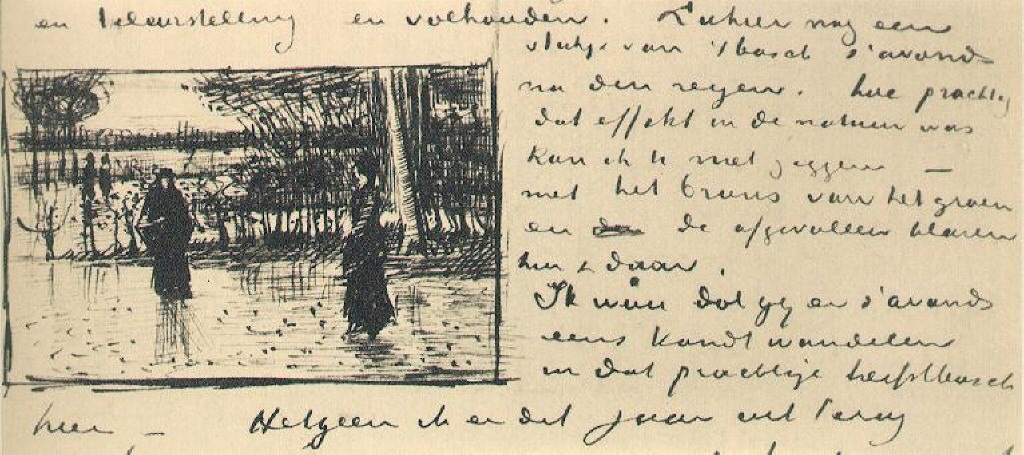The image features an aged, beige paper that gives the appearance of an old handwritten letter, adorned with a detailed pen and ink drawing. Surrounding the drawing, there's a notable amount of cursive text written in black ink, possibly in German, though it's difficult to decipher due to its old-fashioned script. The center-left of the page is dominated by a square drawing depicting two human figures facing each other. Both figures are dressed in long black robes and have their heads covered. The left figure wears a black brimmed hat, while the right figure, partially in profile, appears to have black hair and is dressed in a black dress. The background of the drawing includes roughly sketched trees and bushes, adding a natural, somewhat mysterious ambiance to the scene.